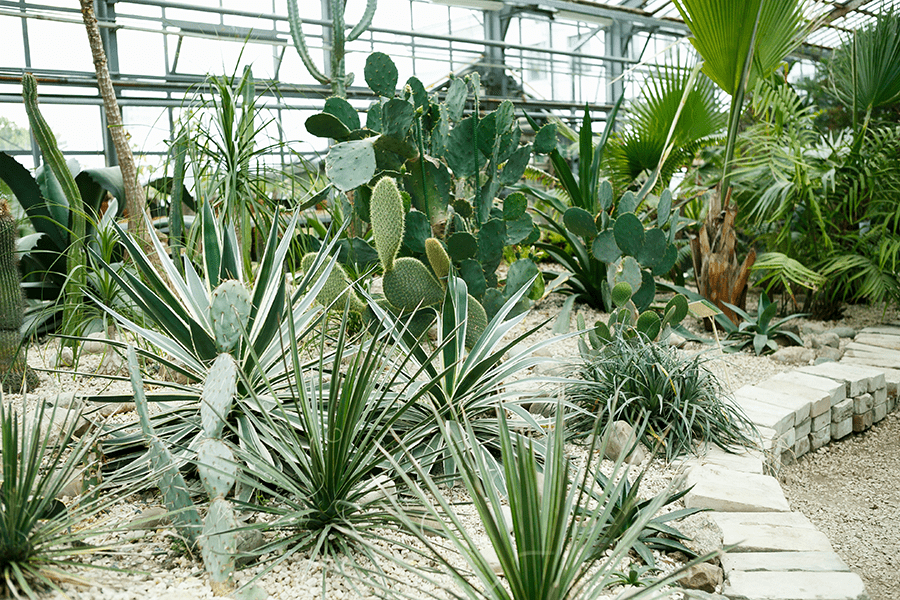This detailed photograph captures the lush interior of a giant glass and metal greenhouse, filled with an array of plants and flowers. The scene showcases a diverse assortment of greenery, prominently featuring various types of cacti and succulents. These plants, differing in size from small to large and including spiny, flat, and oblong cacti, are planted in a gravel-like, whitish soil. On the right side of the image, a path is delineated by stacked gray and white cinder blocks, leading through the verdant display. The greenhouse's structure is visible, with glass windows and metal bars letting abundant light flood in. Additionally, a small sign in the foreground hints at informational content about the surrounding plants, suggesting an educational component to this meticulously arranged plant haven. The overall ambience is one of tranquil, organized chaos with a harmonious blend of nature and architecture.